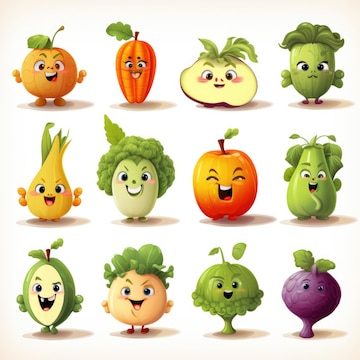This digitally-drawn, cartoon-style illustration features three rows of four anthropomorphized vegetables against a white or off-white background with beige accents. Each vegetable character is rendered in vibrant colors, including orange, green, yellow, purple, and tan, all sporting playful and goofy expressions.

In the top row:
- The first character is an orange, spherical vegetable with a mischievous smile.
- The second is a cheerful orange squash with a green leaf on top, sticking its tongue out.
- The third is a cross-section of an apple with eyes, rosy cheeks, and a smile, looking directly at the viewer.
- The fourth character resembles a cabbage with a closed mouth, stylized shock of green hair, and expressive eyes.

In the middle row:
- The first is a yellow or orange radish with an open mouth, pink tongue, and blushing cheeks.
- Next is a broccoli floret with green hair-like head, smiling mischievously.
- The third appears to be a smiling apple with closed eyes and eyebrows, a stem on top.
- The fourth is an ambiguous green-faced vegetable, either a pear or a green apple, with leaves sprouting from its head and sides.

In the bottom row:
- The first is a green vegetable with a slice taken out, revealing a face missing a front tooth.
- The second is a pale-orange vegetable with leaves on top, smiling brightly.
- The third almost resembles an upside-down cabbage and is also smiling.
- The final character is a bulbous purple vegetable with blended-in eyes but no visible mouth, standing on a pedestal with leaves sprouting from its head.

Each character is depicted with shadows, adding depth to the whimsical, anthropomorphized vegetables, making them appear as if they're engaged in lively conversation or play.